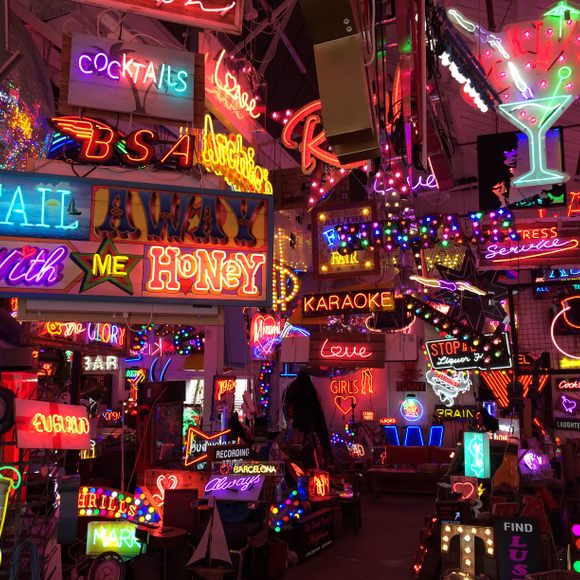The photograph showcases a vibrant, indoor scene filled with an array of neon signs in various colors, including reds, blues, yellows, purples, greens, and pinks, suggesting the inside of a neon sign store or a bar. The image is vertically oriented and teems with colorful lights and signs that convey a lively, eclectic atmosphere. Prominent neon phrases such as "cocktails," "karaoke," "love," "bar," "honey," and "me" are strategically placed, with "love" and "karaoke" featured centrally, "honey" and "me" positioned to the left. Additionally, signs like a giant "R," "stop," and "BSA" in capital letters further enhance the scene's dynamic complexity. A cocktail glass illustration and a star billboard with the word "me" add extra visual interest. A hint of human presence is suggested by the silhouette of a woman who appears to be positioned behind the bar, either placing or collecting an order, adding to the lively social ambiance of the location.